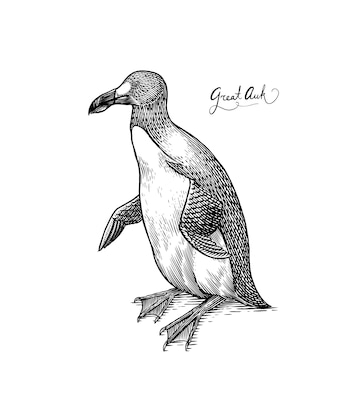This hand-drawn, black-and-white sketch depicts a great auk, labeled in cursive next to the image. The bird, reminiscent of a penguin, features distinctive penguin-like characteristics. It has a short black bill with a prominent white spot, transitioning into darker shades, and is illustrated with fine details that suggest a feathery texture. The great auk is portrayed in a sitting or standing upright position, with its wings lowered but slightly spread open. The bird's white chest and belly contrast with its dark black back, giving it a sense of shading and depth. Its large webbed feet are clearly visible, adding to the creature's detailed appearance.